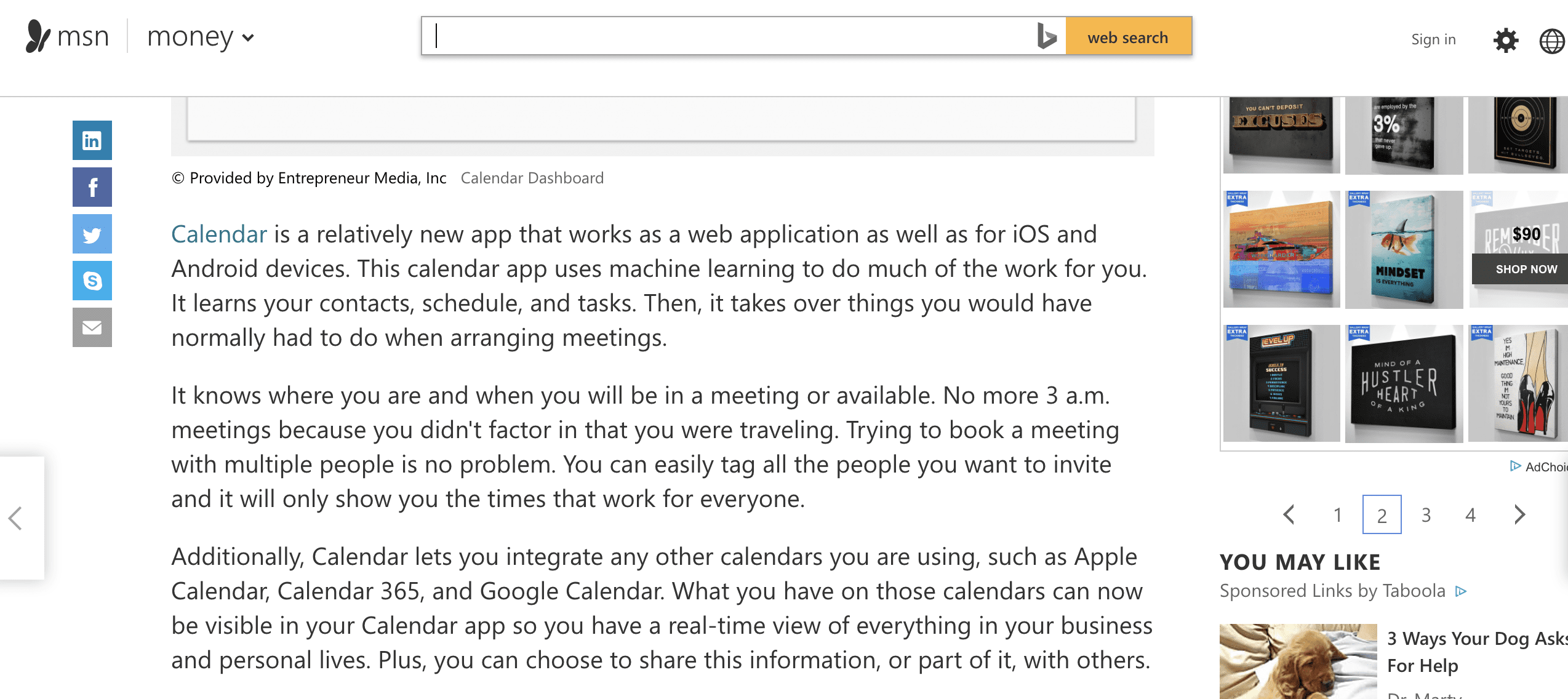This image is a screenshot from the MSN website, showcasing the clean and minimalist design typical of the platform. The background is predominantly white, creating a clear and uncluttered interface. 

In the upper left corner, the iconic MSN logo appears in black, accompanied by the recognizable MSN butterfly emblem. To its right, the section labeled "Money" is displayed with a down arrow, indicating a dropdown menu for financial content. Adjacent to the "Money" section is a search box, ready for user input, followed by an orange button with the text "Web Search" in black. Further right are options to "Sign In," a settings icon, and a world icon, possibly for language or regional settings.

Beneath this header, on the right side, are icons that appear to represent different wall art options. Below these icons is a Taboola advertisement, indicated by the text "You may like: Sponsored Links by Taboola."

On the left side of the screen are icons for various social media and communication platforms, including LinkedIn, Facebook, Twitter, Skype, and email. Directly below these icons is a hyperlink titled "Calendar" in blue. This section introduces a new application called Calendar, which functions as both a web application and a mobile app compatible with iOS and Android devices.

The Calendar app leverages machine learning to streamline scheduling by learning the user's contacts, schedules, and tasks. It automates numerous tasks involved in arranging meetings, such as factoring in time zones to prevent errors like scheduling meetings at 3 a.m. when traveling. The app facilitates booking meetings with multiple participants by displaying only the available times that suit everyone involved. Additionally, Calendar offers integration with other popular calendar services including Apple Calendar, Calendar 365, and Google Calendar, providing a comprehensive, real-time view of all personal and business events. Users can also choose to share some or all of this information with others.

This detailed screenshot encapsulates the user-friendly design and advanced functionalities of the MSN website, particularly highlighting the innovative features of the Calendar application.